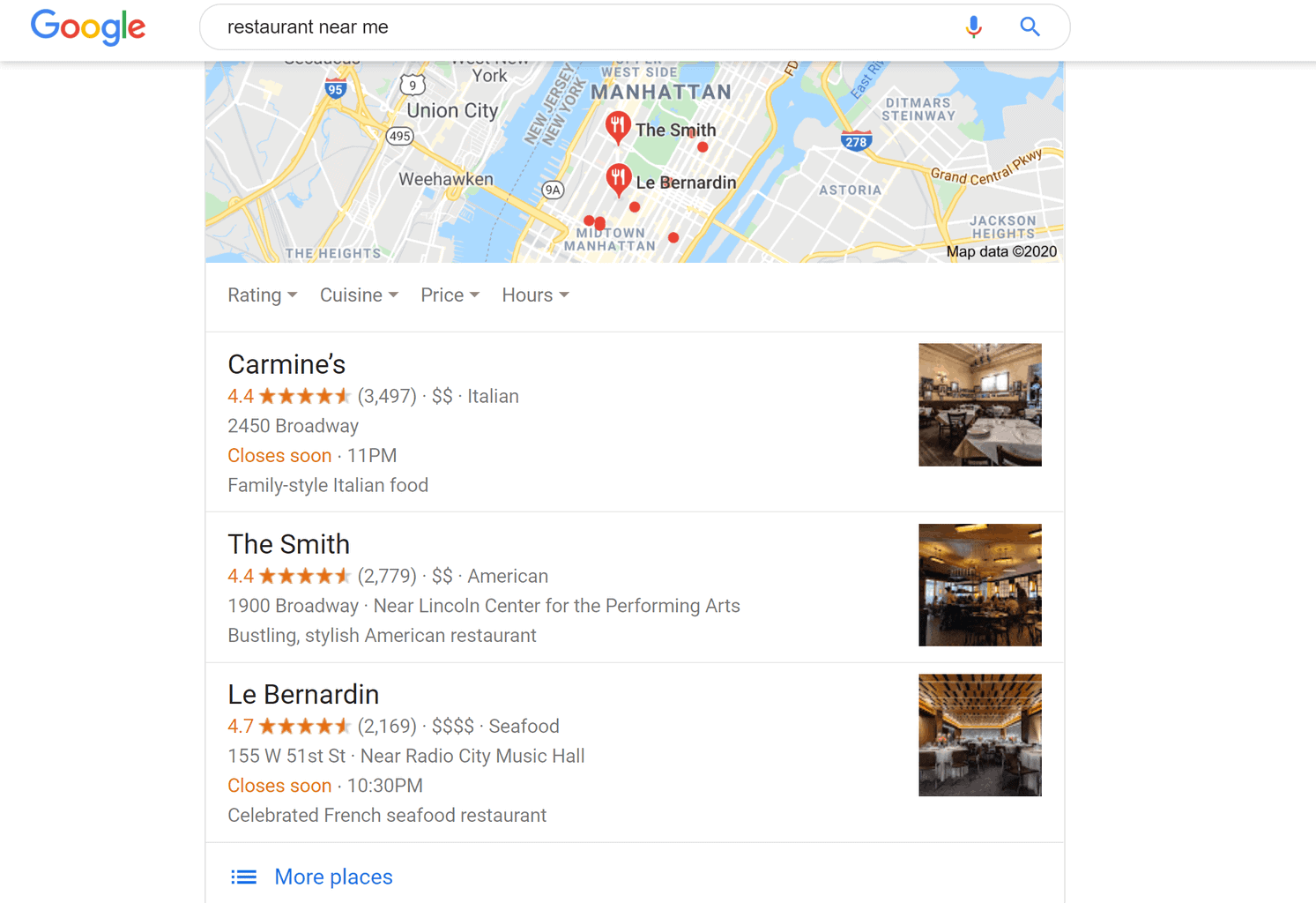This image depicts a detailed Google search result for "restaurant near me," likely from a user in New York City, specifically Manhattan. The top left displays the recognizable Google logo, followed by the search bar where the query "restaurant near me" is entered. Below this toolbar is a small map of Manhattan, highlighting two restaurants with fork and knife symbols.

Underneath the map, three restaurant options are listed:

1. **Carmine's**
   - **Rating:** 4.4 stars
   - **Price:** $$
   - **Cuisine:** Italian
   - **Location:** 2450 Broadway
   - **Closing Time:** Closes soon at 11 p.m.
   - **Description:** Family-style Italian food
   - **Image:** To the right, an interior photo of Carmine's is displayed.

2. **The Smith**
   - **Rating:** 4.4 stars (highlighted in orange)
   - **Reviews:** 22,779 reviews
   - **Price:** $$
   - **Cuisine:** American
   - **Location:** 1900 Broadway, near Lincoln Center for the Performing Arts
   - **Description:** Bustling, stylish American restaurant
   - **Image:** To the right, an interior photo of The Smith is shown.

3. **Le Bernardin**
   - **Rating:** 4.7 stars (highlighted in orange)
   - **Price:** $$$$
   - **Cuisine:** Seafood
   - **Location:** 155 West 51st Street, near Radio City Music Hall
   - **Closing Time:** Closes soon at 10:30 p.m.
   - **Description:** Celebrated French seafood restaurant
   - **Image:** To the right, an interior photo of Le Bernardin is displayed.

Each listing provides a comprehensive view of the restaurant's rating, price range, cuisine type, location, closing time, and a brief description, accompanied by an interior photo for visual reference.